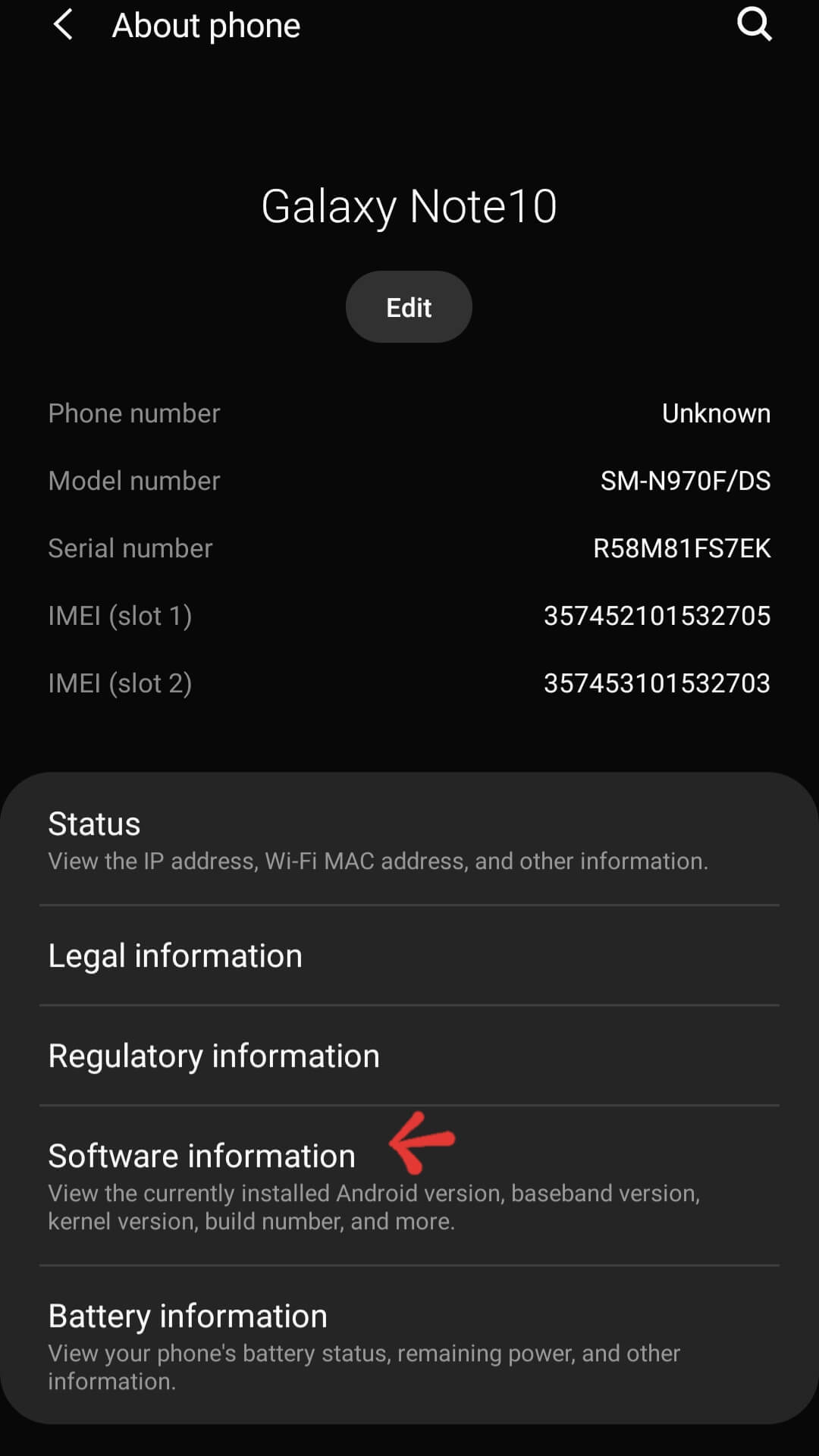This is a detailed screenshot from a Galaxy Note 10 smartphone, showcasing the "About Phone" section. At the very top, on the left-hand side, there's an arrow icon allowing users to navigate back to previous menu options. Adjacent to this is the title indicating the user is in the "About Phone" section. On the right side, a magnifying glass icon is available for searching within the phone’s settings.

Beneath this header is a black background with the title "Galaxy Note 10," identifying the specific model of the device. Below this title is a small gray cylindrical button labeled "Edit." 

The screenshot provides an organized, detailed list of phone information:

- On the left side, in gray text, are categories including Phone Number, Model Number, Serial Number, and IMEI for slots 1 and 2. 
- Corresponding to these categories on the right side are the details: the phone number is marked as unknown; the model number is listed as SM-N970F-DS; both the serial number and IMEI details are displayed as alphanumeric strings for each respective slot.

Further down the page, a gray sequence lists additional information options:

- The "Status" section, which allows users to view the IP address, Wi-Fi MAC address, and other relevant data.
- The "Legal Information" section, followed by "Regulatory Information" and "Software Information." The "Software Information" section is highlighted with a red arrow pointing to it, emphasizing its importance.
- At the bottom is an option labeled "Battery Information," providing details about the device’s battery status.

This comprehensive layout helps users navigate crucial details regarding their Galaxy Note 10 device.